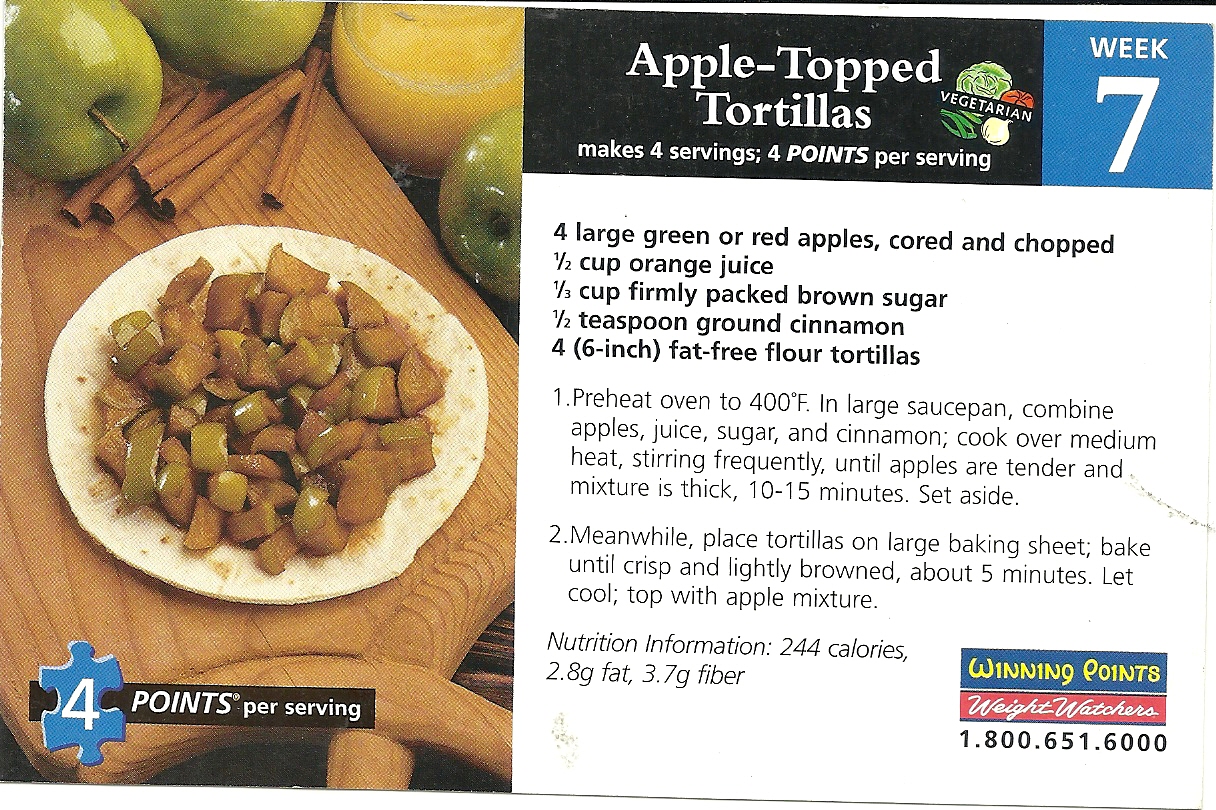This color photograph features what appears to be a recipe card or part of food packaging, likely related to Weight Watchers. On the left side is a photograph of the prepared dish: chopped food in shades of brown and green, served on a white plate. At the top of the plate, green fruit and a glass of juice—possibly orange or lemon juice—are visible. Thin, brown rectangular objects sit alongside the dish, resembling breadsticks or pretzel rods. A blue puzzle piece rests on a wooden board at the bottom, displaying the number "four" in white, accompanied by "points per serving" in white text on a black background.

On the right side of the photograph, towards the top, the dish is labeled "Apple Topped Tortillas," specifying "makes four servings" and "four points per serving." Next to this, a blue square denotes "Week Seven." The black background text to its left contrasts with the adjacent recipe, which is presented on a white background. The recipe details how to prepare the dish, with nutritional information listed towards the bottom.

In the bottom right corner, "Winning Points" is written in yellow on a blue background. Below this, the Weight Watchers logo is displayed in red text on a white background, with a series of numbers that appear to be a telephone number.